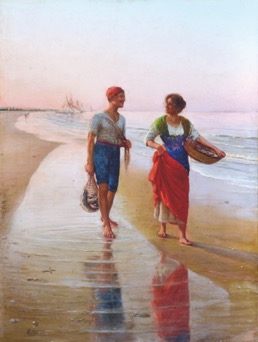The painting depicts two women walking along a beach, each carrying something. The woman on the right side is moving forward, her head turned back towards the other woman on her left. She is barefoot, dressed in a multi-layered outfit including a blue dress, a green scarf over her shoulders, a white shirt, and a red towel wrapped around her waist. She holds a brown basket in her left hand that sticks out to the right. The woman on the left, wearing a red bandana, a white shirt with sleeves ending just above her elbows, and blue knee-length shorts, is walking through a puddle of water. She carries a net or a bag that appears to contain fish in her left hand. The beach scene features water on both sides of the women, with the ocean visible to the far right, light blue with some ripples and transitioning to a whitish color further back. The sky above is a gradient from light blue to pink, indicating sunset. A dead bush or tree with a few branches can be seen along the horizon line in the background. The reflections of the women, specifically the red towel and the person in the puddle, are visible in the rippling water below them.